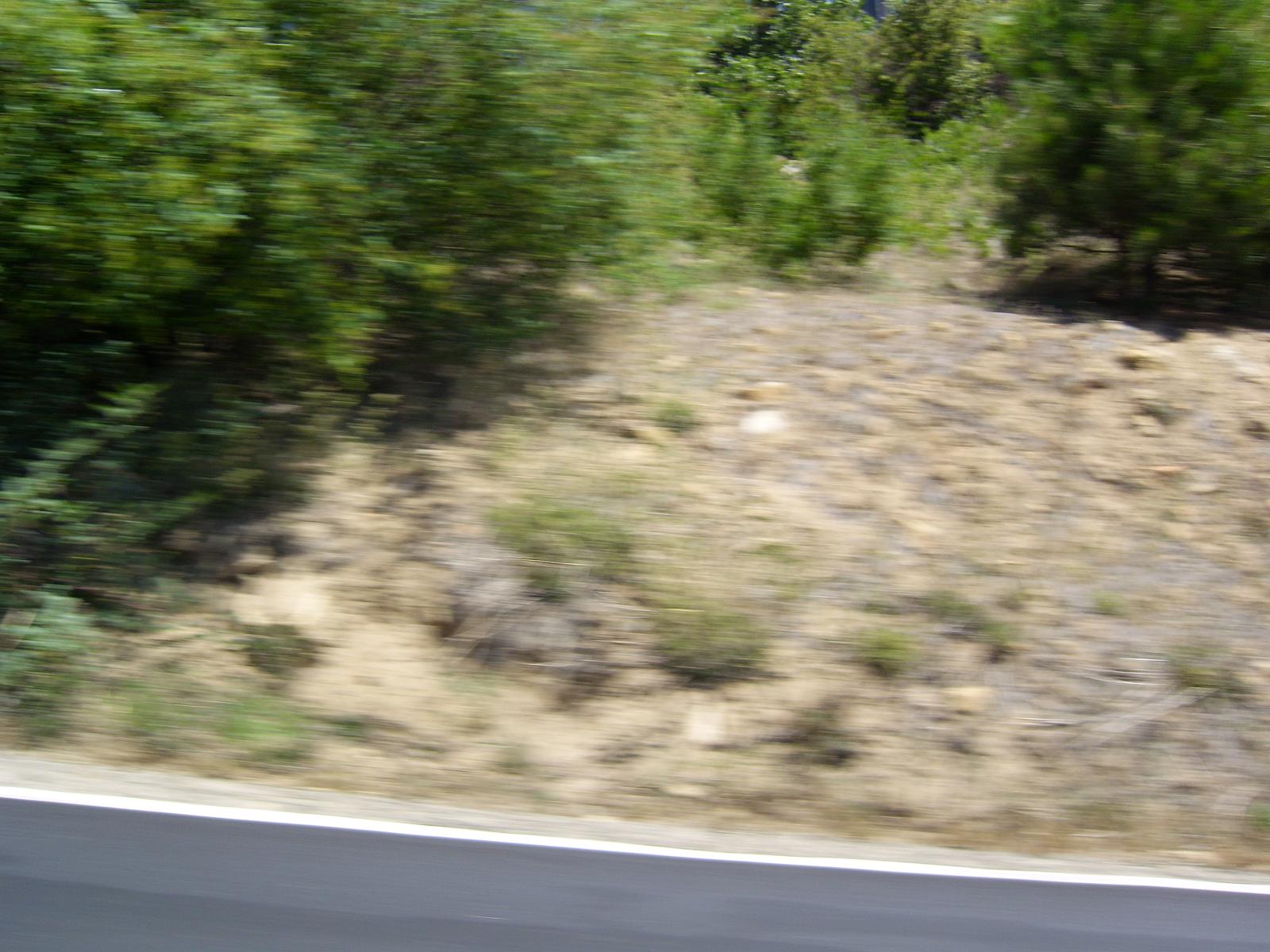This blurry, landscape-oriented photograph captures an outdoor scene during daytime. The image is taken possibly from a moving vehicle, evident from the slight motion blur affecting the overall focus. In the foreground, there is a patch of grey asphalt, indicative of a road, with varying shades of grey and a white lane marking running through it. Beyond the road lies a yellowish, gravelly bank common to rural highway shoulders, interspersed with patches of desert-like sand and scrubland.

To the left and extending upwards into the background, patches of green are visible as foliage and bushes, along with trees exhibiting leaves in various shades of green, from dark to light. A specific object, perhaps the size of a tennis ball and white in color, is nestled among the gravel, though the blurriness makes it challenging to discern whether it is a rock, a piece of litter, or another item. The entire scene, characterized by brown and green hues with some splashes of grey, presents a snapshot of a roadside environment, framed by nature in a state of slight disarray.